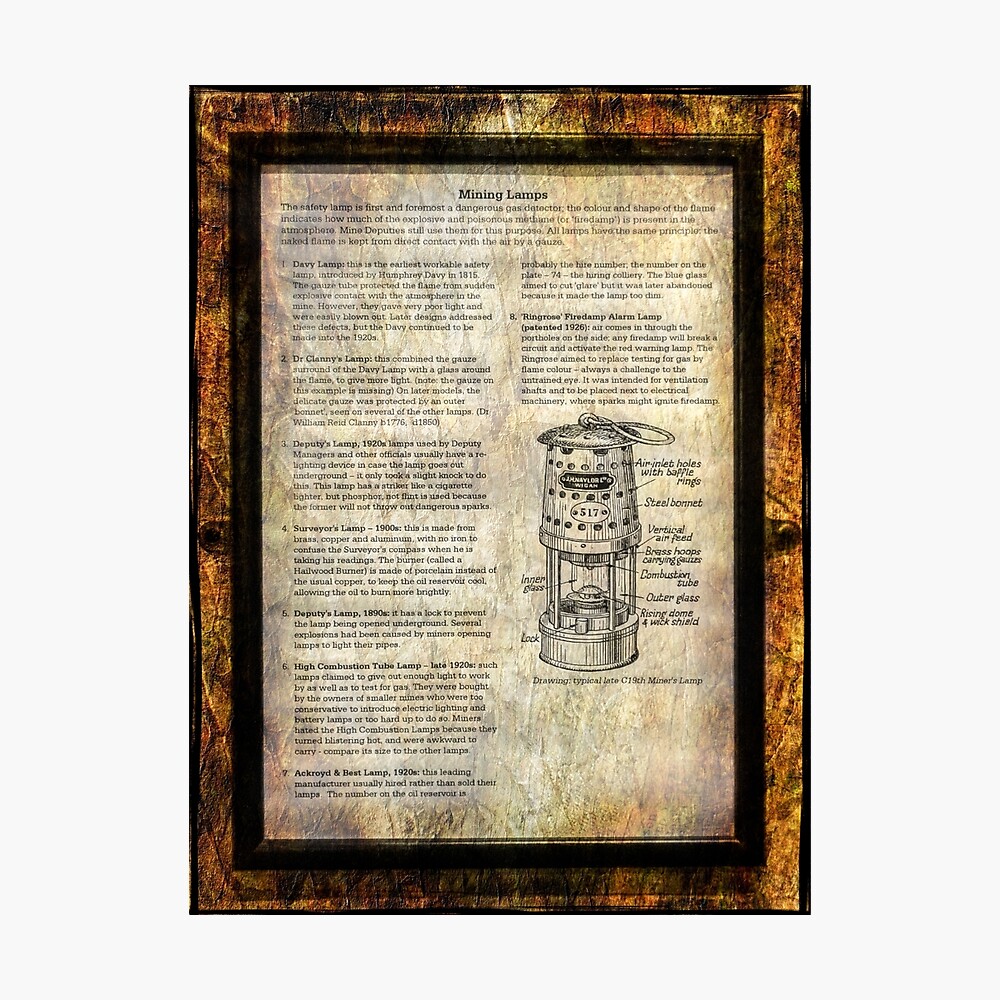This image features a framed, pen-and-ink illustration set against a soft, very light gray background and surrounded by a golden speckled frame. The artwork itself is rendered on a light yellow, somewhat shiny and textured paper, and details a comprehensive guide to mining lamps. At the top of the page, the title reads "Mining Lamps" in prominent black text. The diagram within the frame meticulously labels and explains the various parts of a mining lamp, emphasizing its key role as a dangerous gas detector. The text runs along the left and top right sides of the illustration, providing eight detailed instructions on how to use the lamp safely. Additionally, the central section of the image features explanations and historical context about these lamps, tracing their evolution from the 1800s to the 1920s. This detailed illustration could easily be an informational kiosk or signage found in a museum, offering an educational overview of mining lamps and their components, such as the outer glass combustion tube.